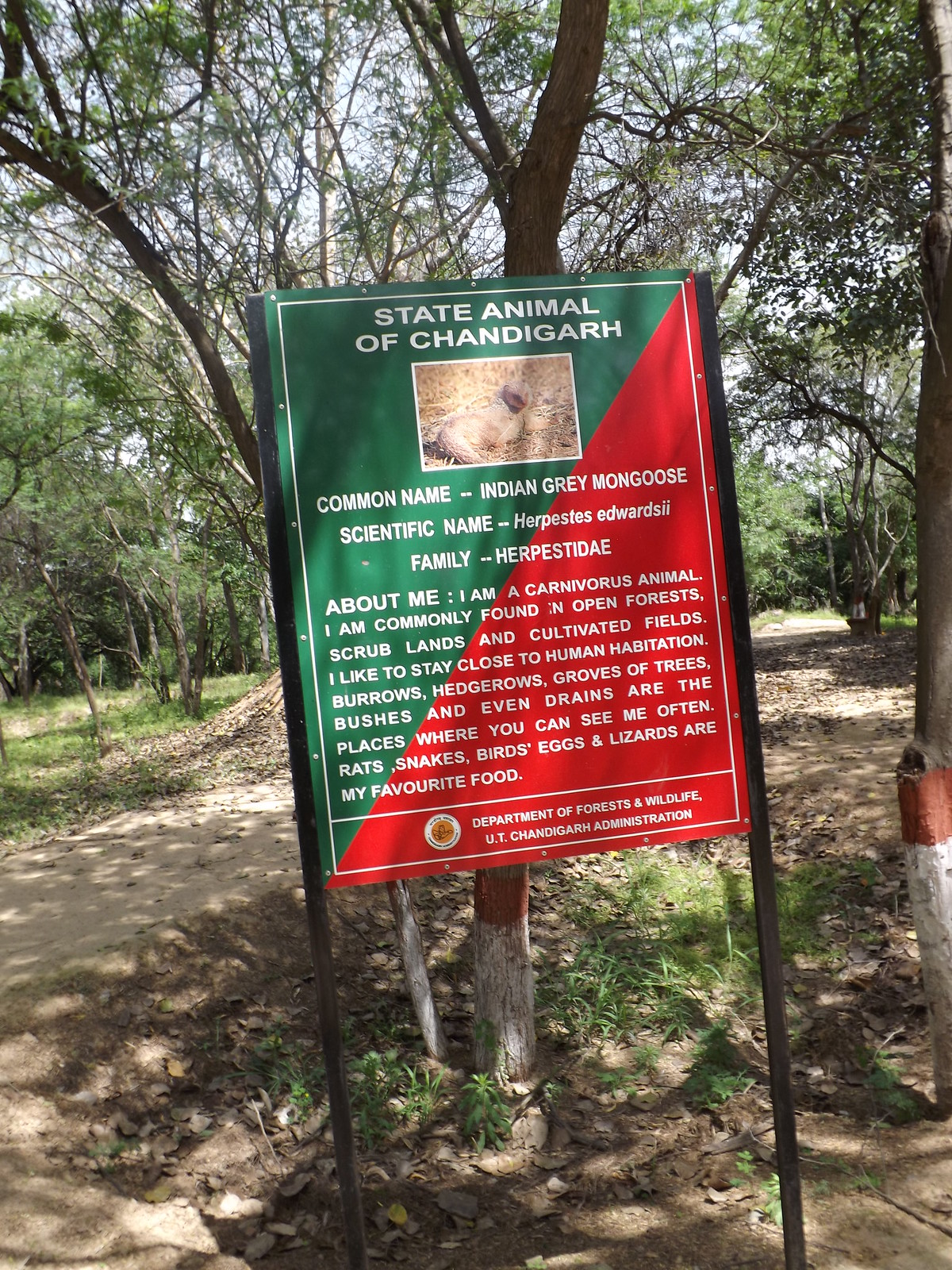The image captures an outdoor scene in a park, featuring a dirt trail meandering through a lush, tree-dense area with green foliage. Sunlight filters through the canopy, casting dappled light and creating a serene atmosphere. Prominently displayed in the foreground is a rectangular sign, mounted on black metal posts that are firmly embedded in the ground. The sign is divided diagonally, with the upper half in green and the lower half in red, and features white text. At the top, it reads "State Animal of Chandigarh" and below that, it includes a photograph of an Indian Gray Mongoose on brown grass, bordered in white. The sign provides further details with the common name "Indian Gray Mongoose," its scientific name "Herpestus edwardsi," and its family "Herpestidae." Additional information about the mongoose explains its carnivorous diet and habitat preferences, mentioning its presence in open forests, scrublands, cultivated fields, and near human habitation, including burrows, hedgerows, groves of trees, bushes, and drains. The text notes that its favorite foods are rats, snakes, birds, eggs, and lizards. At the bottom of the sign, the authority is credited as the "Department of Forests and Wildlife, UT Chandigarh Administration."